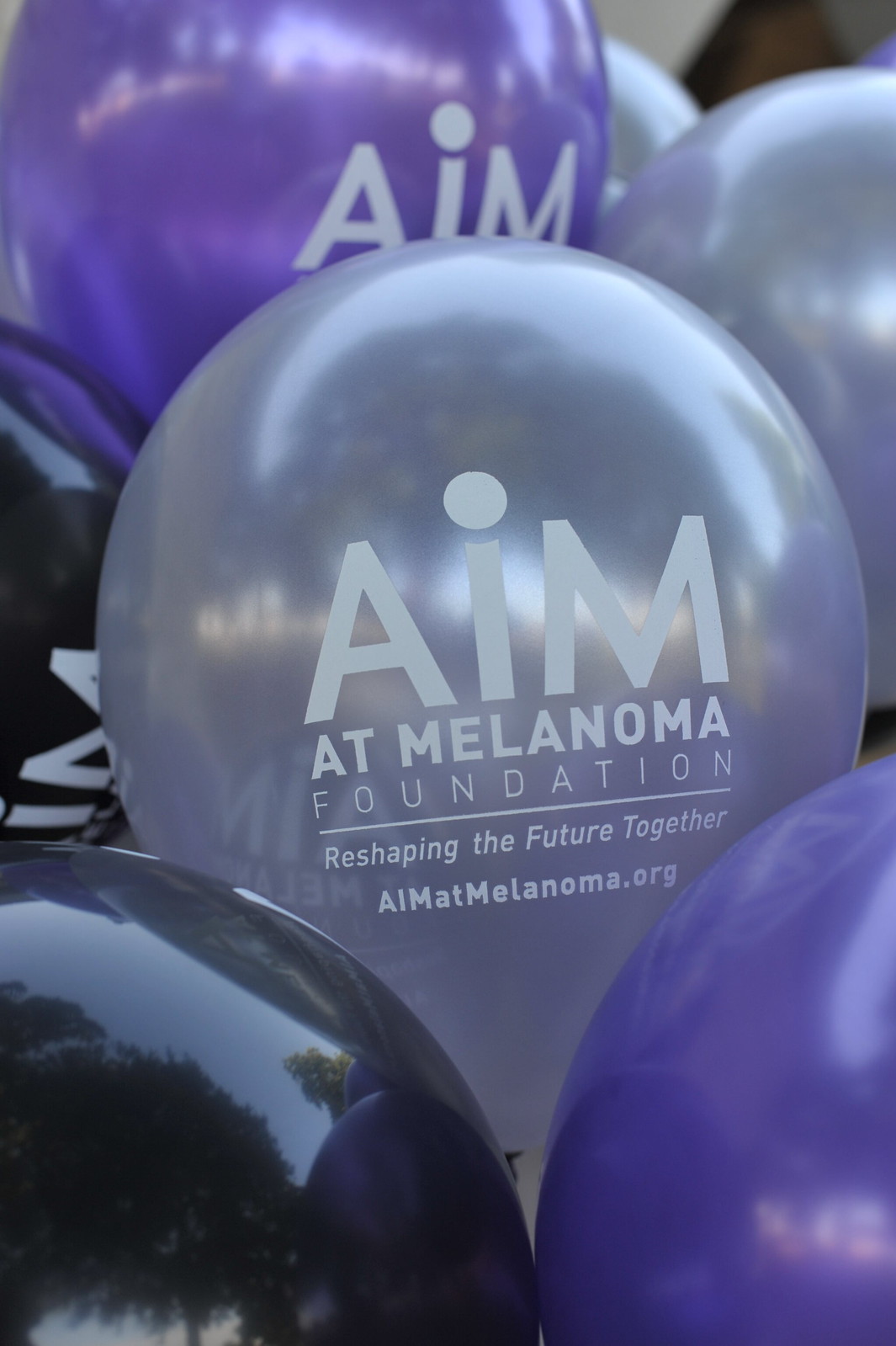This image displays a vibrant arrangement of balloons in various shades of purple, silver, and black, gathered together, with one predominant silver balloon at the center. Each balloon features identical white text: a prominent "AIM" in bold font, followed by "at Melanoma Foundation" in smaller letters. Beneath this, a horizontal line distinguishes the phrase "reshaping the future together," alongside a website link, "AIMatMelanoma.org." The central silver balloon stands upright, surrounded by other balloons in different positions, creating a dynamic and eye-catching scene. The display appears to be part of a charity event or fundraiser, highlighting the efforts of the AIM at Melanoma Foundation to fight skin cancer and promote awareness.